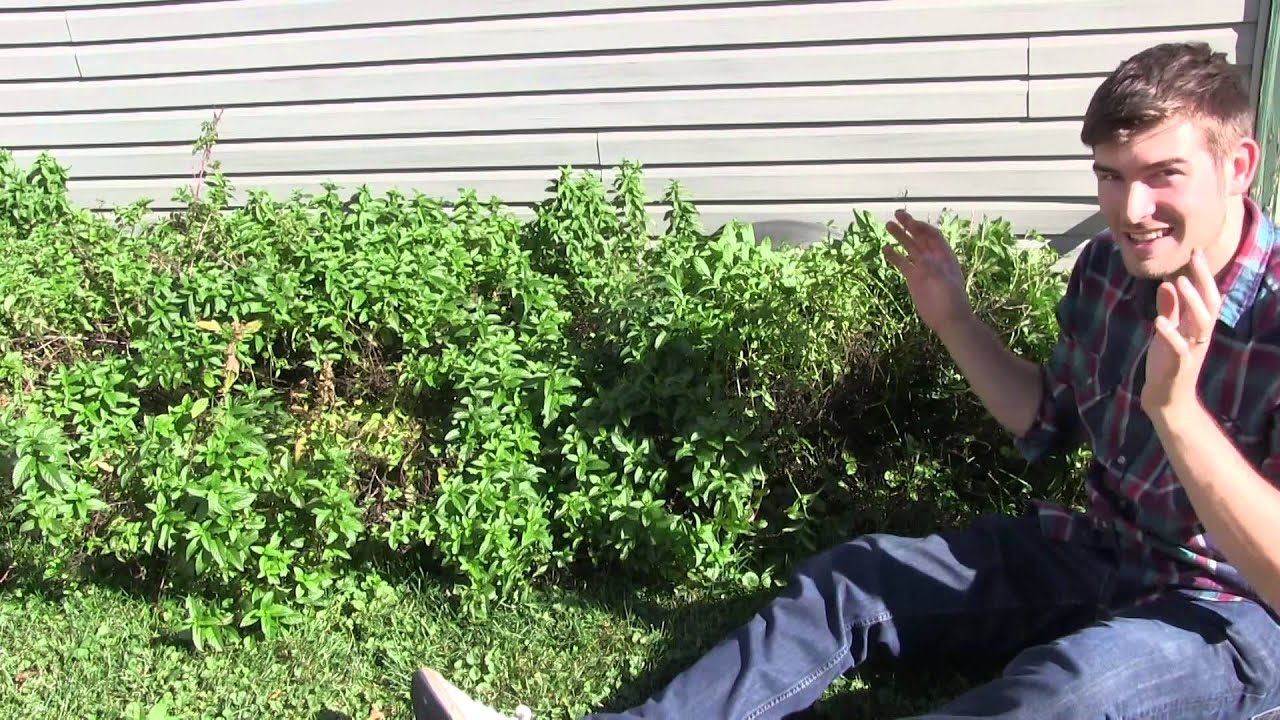This photograph captures a cheerful young man sitting on the ground next to a row of tall weeds or shrubs in a yard. The various shades of green in the grass, weeds, and shrubbery frame the right side of the image, with the man positioned on the far right. The background reveals the lower portion of a house with beige or light-gray horizontal siding. The bright sunlight illuminates the scene, casting light on the man's face. He has light skin, short brown or dirty blonde hair, and is smiling widely, showing his teeth. His hands are raised in front of him, palms open, resembling a playful "jazz hands" gesture. The man is dressed in a plaid flannel shirt with colors including blue, red, and possibly purple, with the sleeves rolled up to his elbows. He also wears blue jeans and white tennis shoes, with his legs stretched out in front of him. The overall ambiance suggests a sunny, carefree moment, perhaps in the man's garden or yard.